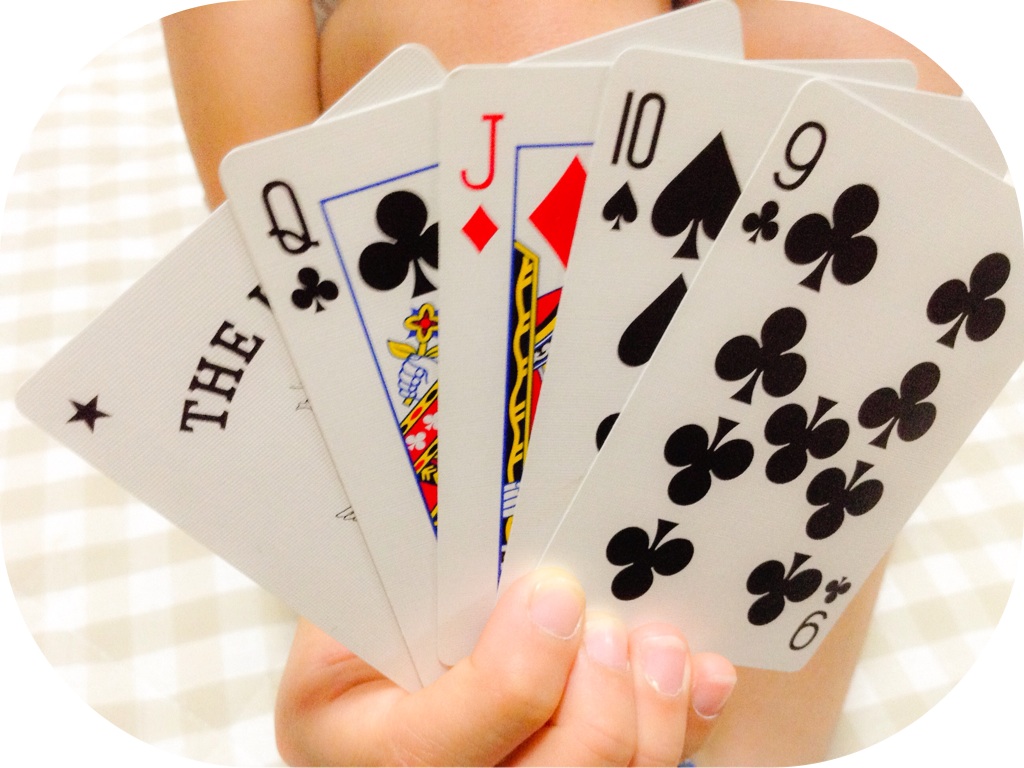In this image, a person’s hand, with short fingernails, is tightly clutching five playing cards. From left to right, the cards displayed are a wild card featuring the word "the," a Queen, a Jack, a Ten, and a Nine. The background reveals some skin, indicating the cards are being held in front of a knee. Below the hand, there is a white and tan crisscross-patterned tablecloth or blanket, adding a cozy and casual atmosphere to the scene.